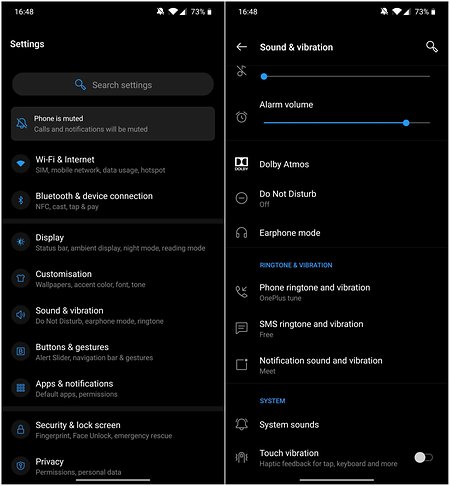The image depicts a screenshot of a phone app's settings interface, specifically focusing on the "Sound and Vibration" section. At the top of the settings menu, various options are visible including "Phone is muted," "Wi-Fi and Internet," "Bluetooth and Device Connections," and more. The current screen highlights the "Sound and Vibration" settings, showcasing various adjustable sliders and toggles. 

In detail, the screen displays:
1. A music volume slider
2. An alarm volume slider
3. An option for Dolby Atmos
4. A "Do Not Disturb" mode toggle
5. An "Earphone Mode" section
6. A "Ringtone and Vibration" section with sub-options such as "Phone Ringtone and Vibration," "SMS Ringtone and Vibration," and "Notification Sound and Vibration"

Each of these sections provides customizable options for the user to adjust the sound settings on their device to their preference.